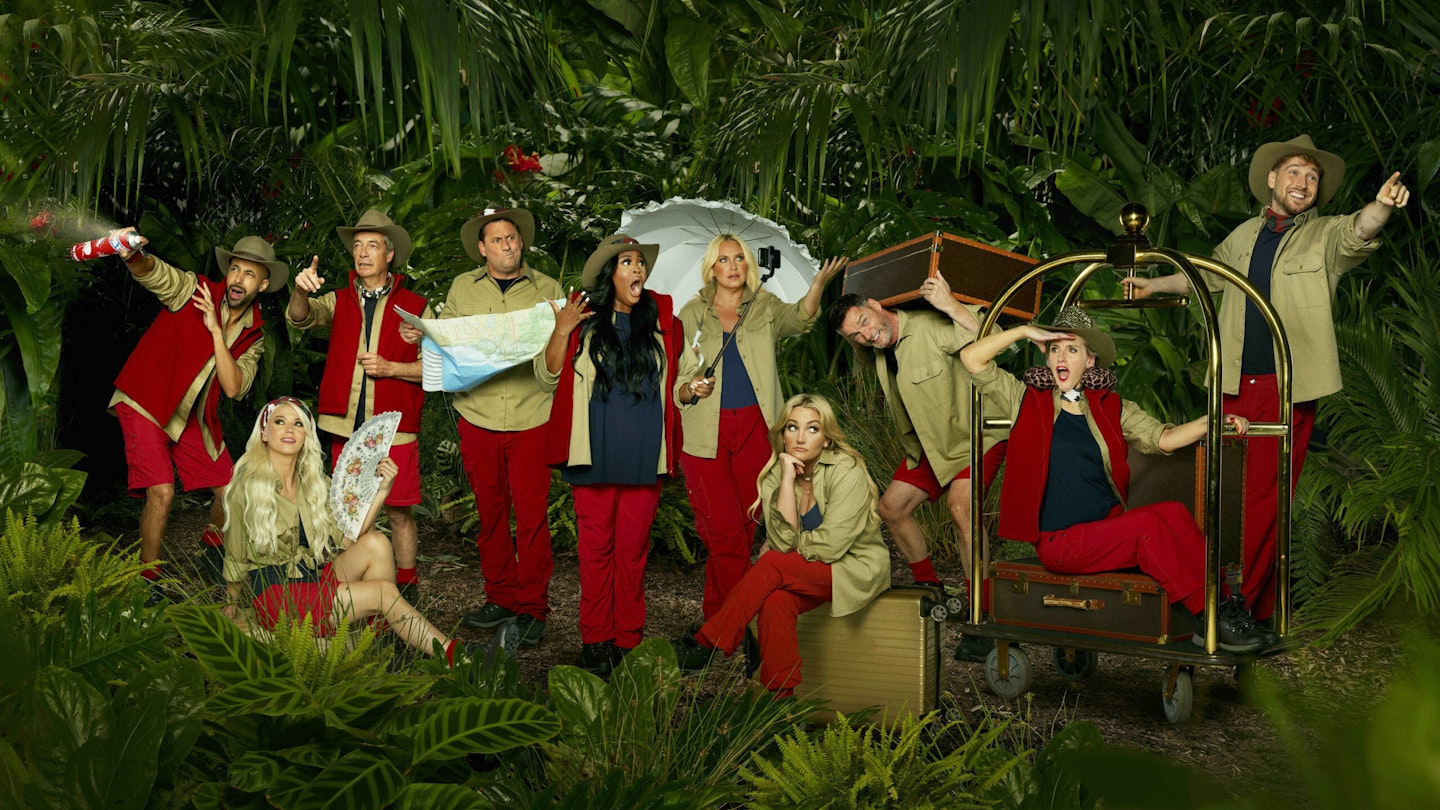In this vividly staged and colorful outdoor photo set against a lush jungle backdrop of palm fronds, ferns, and broadleaf tropical plants, a group of ten travelers, predominantly Caucasian with one black woman, are portrayed in a mix of tan, black, and dark red safari-style outfits. Each person engages in unique activities, suggesting they are stranded travelers. The gentleman on the far left sprays bug spray into the air, while a blonde woman with a white parasol and selfie stick captures the moment. Another woman fans herself with a white lace flag, and a man with a brown hat appears to be consulting a map with a confused expression. Amidst the scattered luggage, another gentleman carries a suitcase on his back and a luggage trolley carries a woman shielding her eyes, seemingly searching for something ahead. Despite the challenges, the group maintains a sense of humor, making silly and cute faces, contributing to the whimsical and adventurous atmosphere of the scene.